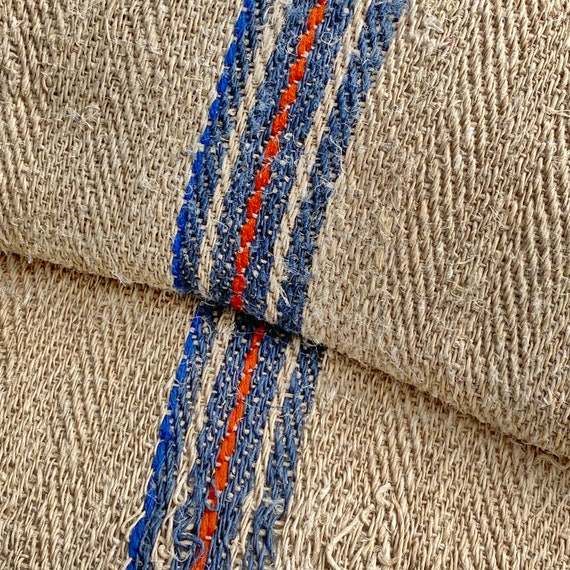This close-up image in color captures a folded piece of fabric that closely resembles burlap with a rough, interwoven texture. The material is naturally tan or light beige, emphasizing its organic look. Prominently featured is a noticeable horizontal fold running from the left to right, creating a section with a striped pattern. This pattern consists of two vertical blue lines on either side. Between these lies a wider blue stripe, highlighted by a thinner red stripe running down its center. The fabric stands out with its thick, coarse weave, adding to its rustic appearance. The image is tightly framed on the fabric, without any background distractions, highlighting the detailed textures and colors.